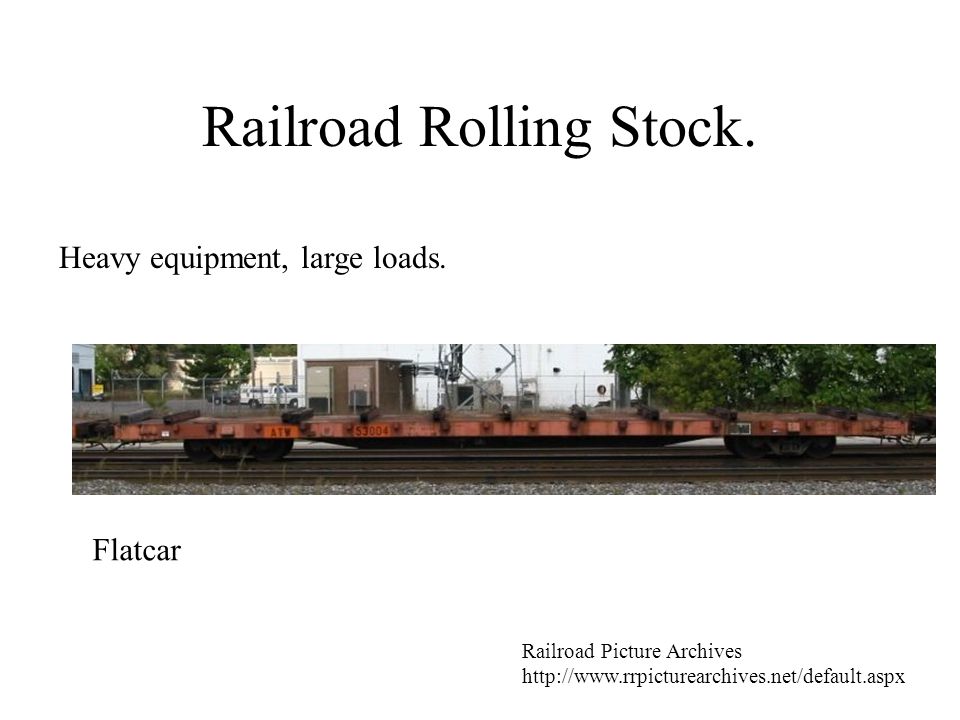The image caption reads "Railroad Rolling Stock" in large Times New Roman font, followed by a smaller text, "Heavy Equipment, Large Loads." The photograph depicts a long, horizontal flatbed railroad car in a rusty orange hue, with black, barely discernible wheels, set on brown train tracks surrounded by gravel. The flatbed railcar has several knobs or spacers and lacks sidewalls or a top. In the background are green trees, a chain-link fence, a white industrial building with parked cars including a white truck, and a cream-colored building. Below the photograph, the text "Flat Car" appears on the bottom left, while "Railroad Picture Archives" and a URL, "http://www.rrpicturearchives.net," are at the bottom right.